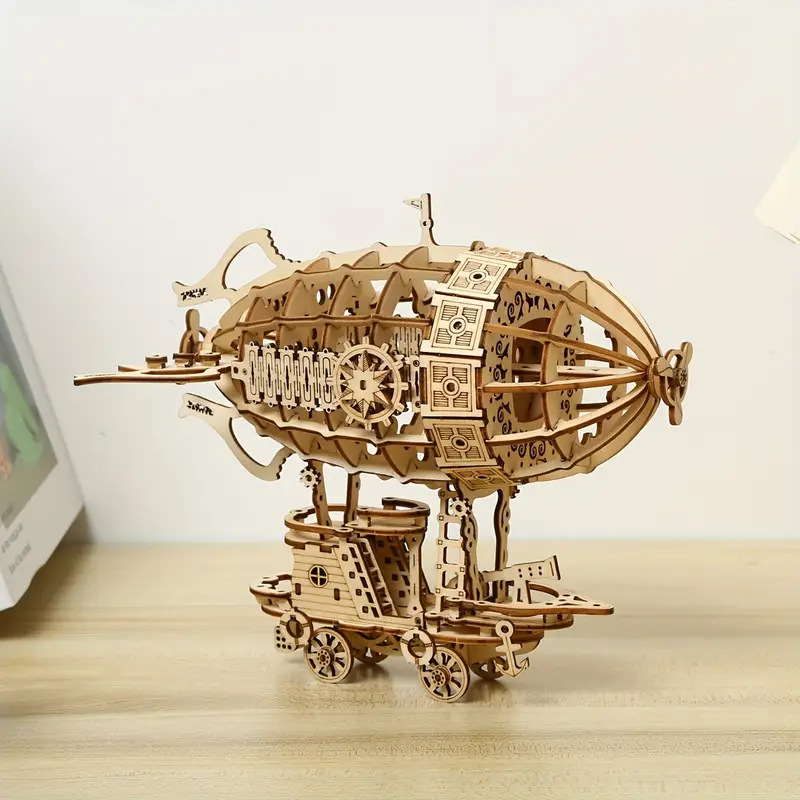This photograph captures a meticulously crafted wooden model set against a plain white wall on a pine-colored tabletop. The model exemplifies a steampunk, fantasy-style vehicle, blending elements of a blimp and a carriage. The blimp, detailed with intricate burned and engraved patterns, boasts propellers at both the front and back, and is supported by large bracers or rudders on the top, bottom, left, and right, suggesting a complex control mechanism. Ornate features include a flag at the top and visible interior details through its open design. The blimp sits atop a four-wheeled wagon, reminiscent of a houseboat on wheels, complete with an anchor, indicating its multi-purpose nature for both air and land travel. To the left of the model, a book with a white cover rests on the tabletop, adding a sense of scale and context to the scene.